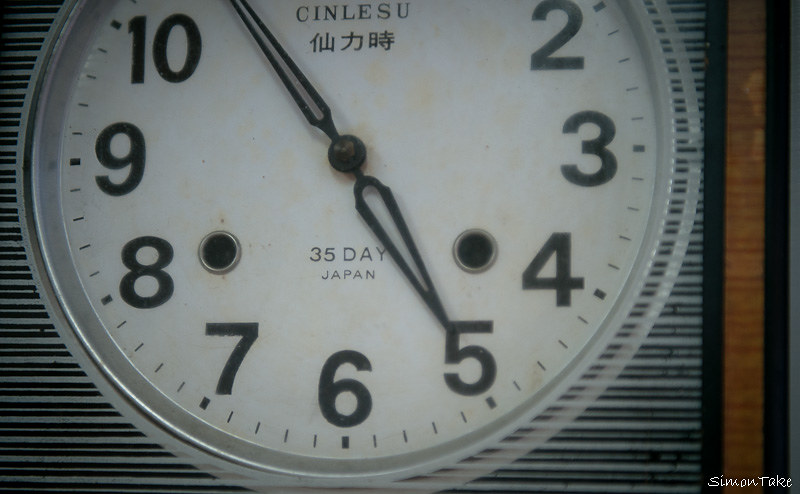In the image, a large, weathered clock with a white face and prominent black numerals is prominently displayed, possibly outdoors. The clock features Japanese writing, including "35 Day Japan." The hands of the clock are transparent, allowing the face of the clock to be visible through them. The clock is set against a striking black and white striped background. On the right side of the image, a vertical strip of wood is flanked by black sections. In the lower right-hand corner, the name "Simon Tate" is visible.